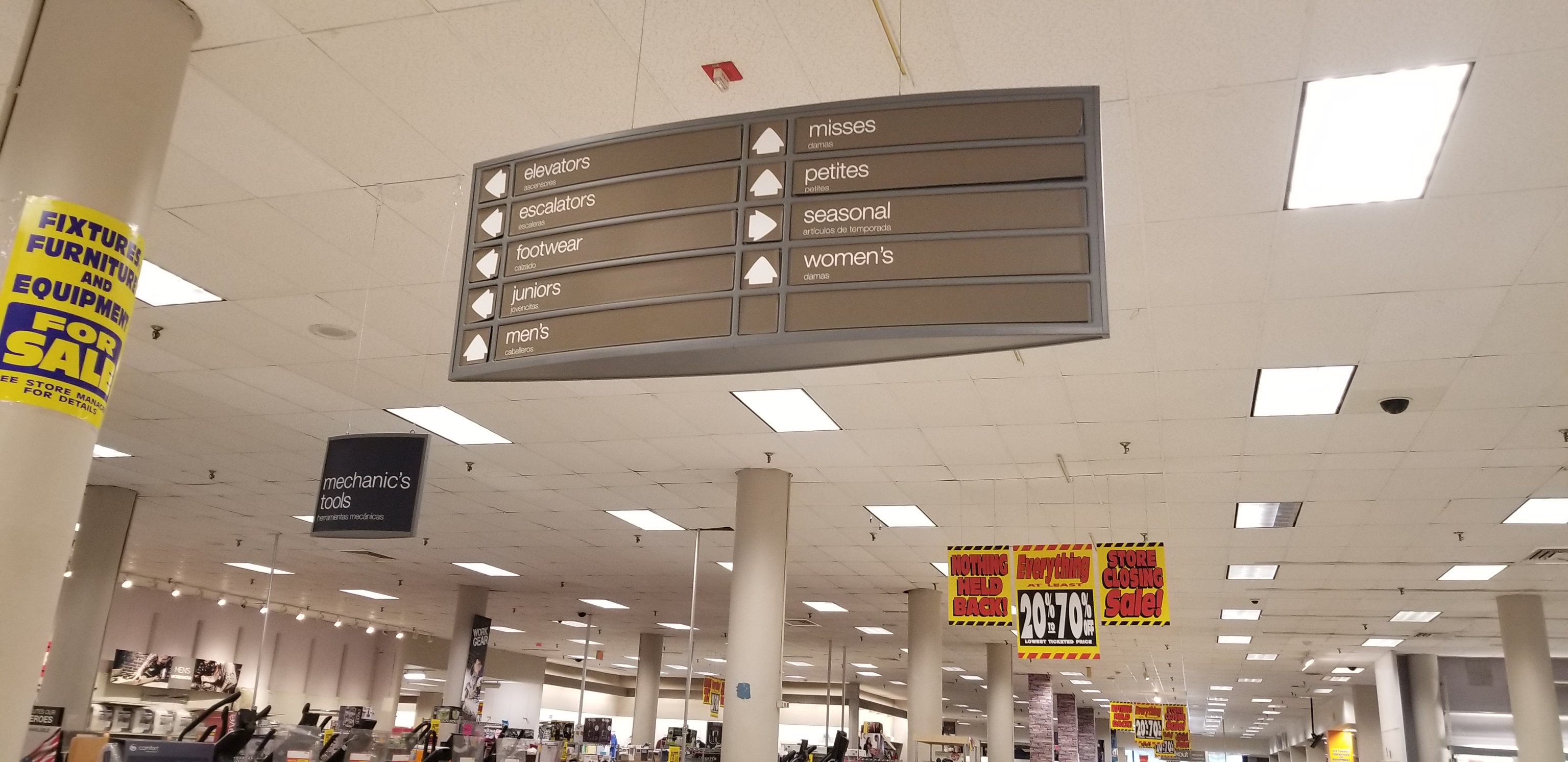The image captures the interior of a retail store reminiscent of a former Sears location, complete with a drop ceiling supported by large columns. On the left side, a variety of lawnmowers are displayed, while further down the aisle, the backs of televisions and possibly other appliances are visible. The center and right sections of the store are filled with large boxes. Signs hung from the ceiling announce a store closing sale, boldly advertising discounts of 20-70% off with the message "Nothing Held Back" repeated throughout the space. Another sign on a nearby column declares "Fixtures, Furniture, and Equipment for Sale." Above the lawnmower display, a sign indicates the area for 'Mechanic's Tools.' Prominent directional signage in the middle of the store points customers to elevators, escalators, footwear, junior men's, Mrs. Petite's, seasonal, and women's sections. Security cameras are installed in the ceiling, documenting the store’s final days. The overall atmosphere is somber, reflecting the end of an era for this once bustling retail outlet.